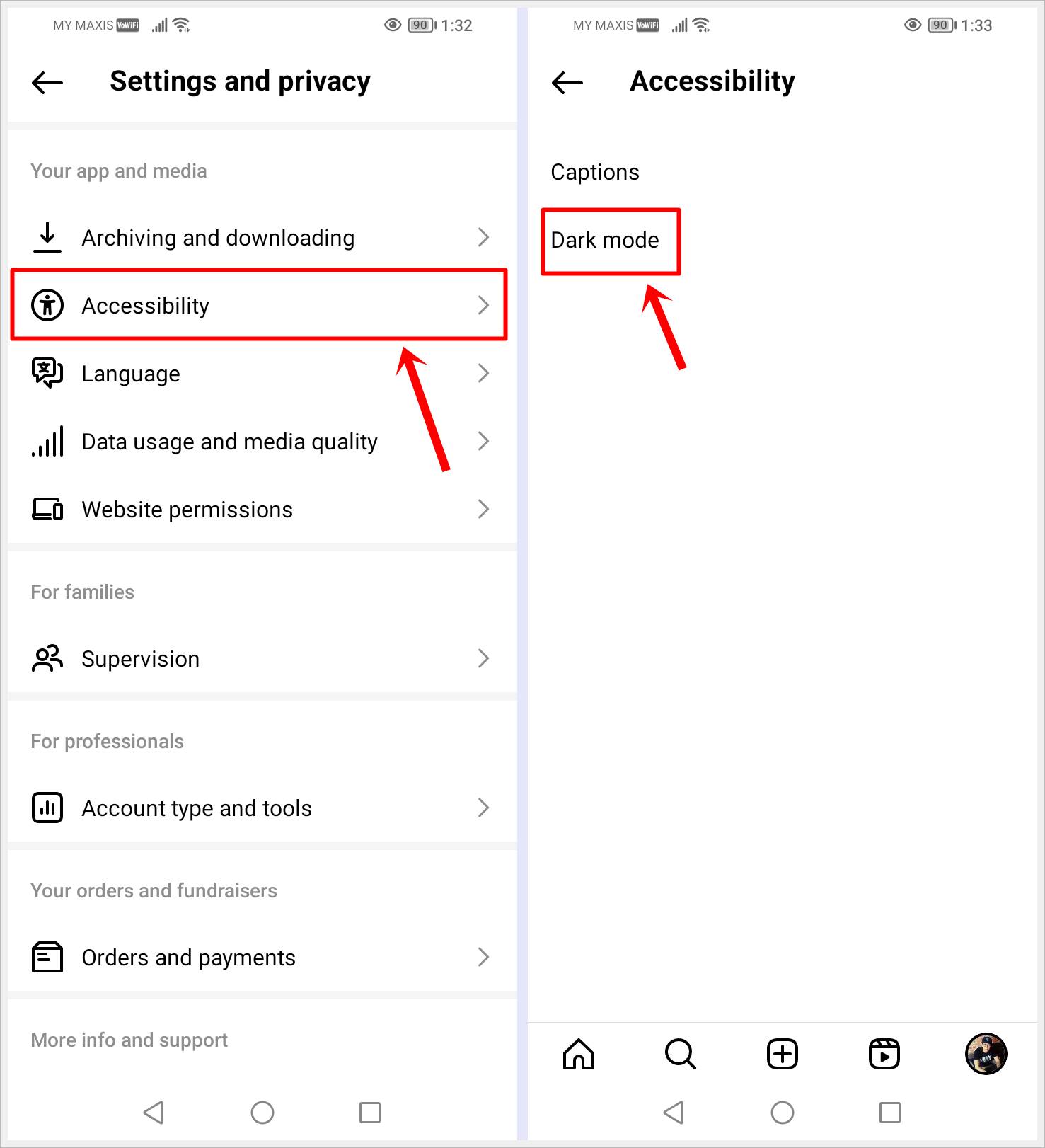The visual highlights the settings interface of an Android application, displaying instructions to access a specific menu option. The image is divided into two side-by-side screenshots taken from an Android device, as indicated by the presence of the standard Android navigation icons: the back arrow (triangle pointing left), home button (circle), and recent apps (square).

Both screenshots are titled "My Maxis" at the top, suggesting the app is likely from a cellular service provider. The status bar displays a strong cellular signal with five bars, full Wi-Fi signal with six bars, a notification icon resembling an eye, a battery level of 90%, and timestamps of 1:32 PM and 1:33 PM respectively for the left and right screenshots.

In the left screenshot, the highlighted heading is "Settings and Privacy," listing several sub-menu options:
1. Your App and Media with a dropdown arrow.
2. Archiving and Downloading.
3. Accessibility (this option is highlighted with a red square and an arrow pointing to it).

Additional options on this page include:
- Language, denoted by a speech bubble with various symbols inside.
- Data Usage and Media Quality, represented by a cellular signal icon.
- Website Permissions.
- For Families, illustrated with two character icons.
- Supervision for Professionals, indicated by a square with lines.
- Account Type and Tools.
- Your Orders and Fundraisers, depicted with a box and labeled Orders and Payments.
- More Info and Support at the bottom.

The right screenshot focuses on the "Accessibility" menu, showcasing two options: "Captions" and "Dark Mode." The "Dark Mode" option is highlighted with a red square and an arrow pointing to it, indicating it's the selected feature.

In summary, this image tutorial demonstrates the process of navigating through the settings of the "My Maxis" app on an Android device to enable Dark Mode via the Accessibility menu.